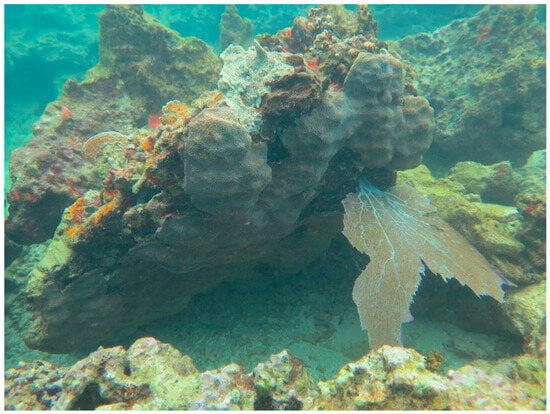This underwater photograph captures a vibrant coral reef, likely situated in an aquarium or a natural seabed too expansive for a simple fish tank. The scene is bathed in a teal hue due to the water, lending an ethereal blue-green tint to everything. The seafloor is layered with light brown, greenish rock formations, and patches of white sand faintly tinged with teal.

Dominating the upper left quadrant of the image is a substantial mass of rock and coral, distinguishable by its light brown underside and vivid growths of orange and reddish algae. This coral structure seems elevated on one side, creating an impression as if it were lifted or toppled, revealing the fine details and holes that scar its surface. Jagged and sharp, this reef is interspersed with barnacles and other circular formations, highlighting its rugged texture.

To the right of the scene, a flat, copper-colored structure that resembles a leaf adds another layer of complexity to the environment. The water surrounding these formations appears murky, with high turbidity that modulates its color to a greenish-blue, enhancing the undersea ambiance of this captivating marine ecosystem.